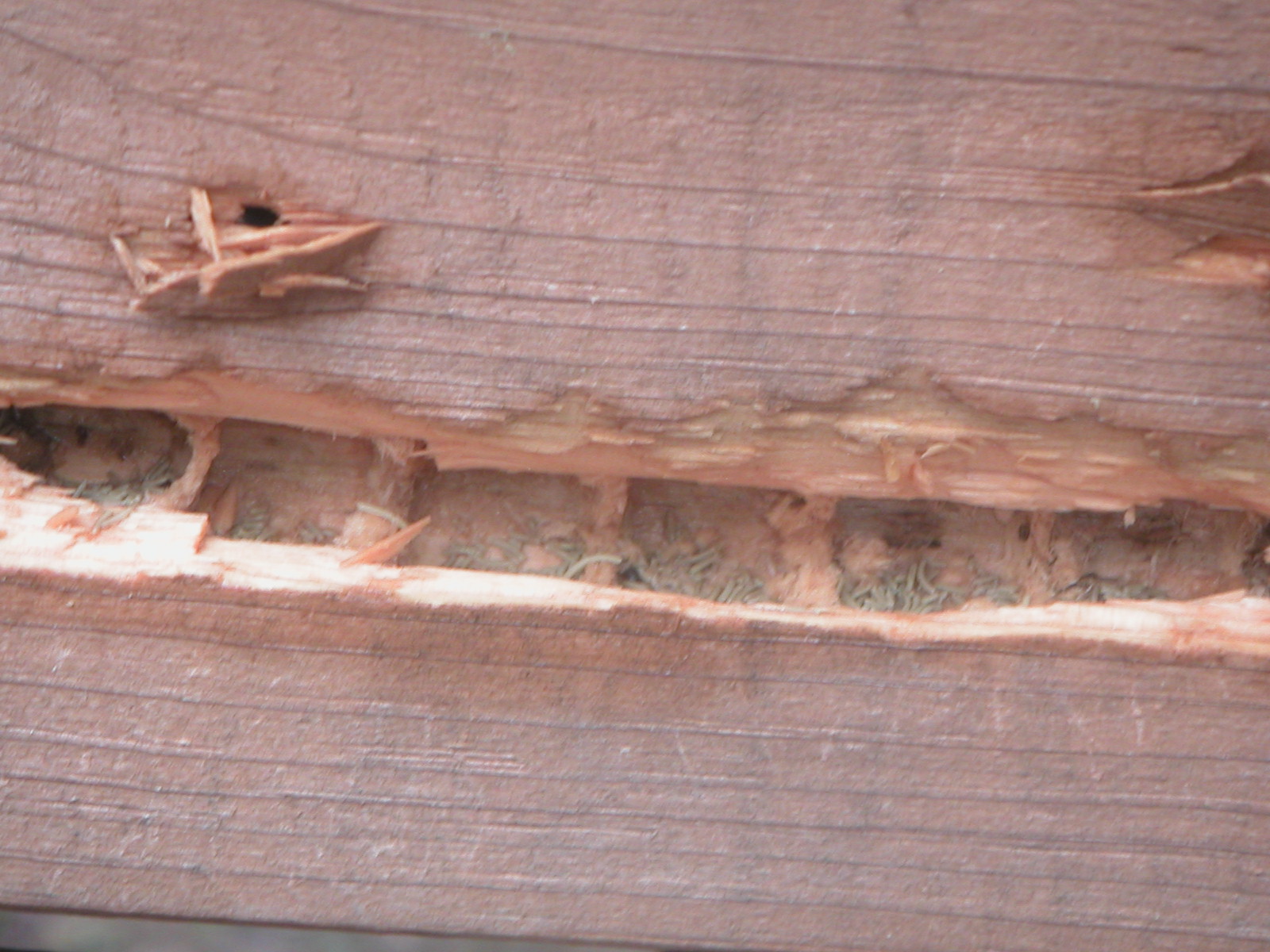This up-close photograph captures a severely damaged plank of wood, likely suffering from insect infestation. The wooden board displays a reddish-brown hue with a slightly pinkish tint and appears rotted and extensively chewed up. Down the center, a prominent section follows the grain and has been gouged out, revealing the inner layers of the wood. Various small, elongated, and light beige-gray larvae are conspicuously visible within the damaged area. These worm-like insects, lacking any visible feet or wings, seem to be responsible for hollowing out the wood. Numerous channels run vertically through the board, each harboring clusters of these larvae, suggesting a heavy infestation that has significantly contributed to the deterioration of the wood.